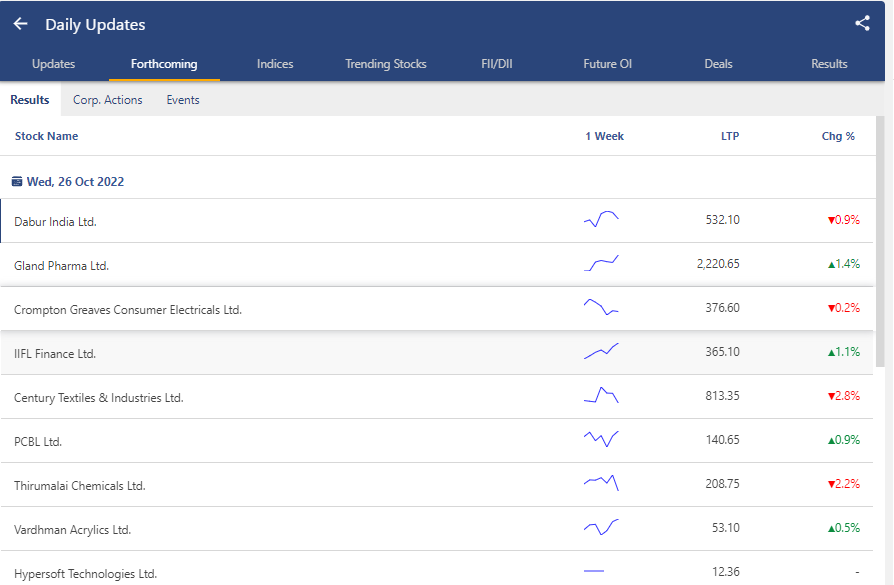The image is a screenshot of a financial website displaying various stock performance metrics and updates. Dominating the top section of the webpage, a large blue rectangle spans across its width with the words "Daily Updates" prominently displayed in white text. Beneath this header, several categories are listed including "Updates," "Forthcoming Indices," "Trending Stocks," "FII-DII," "Future OI," "Deals," and "Results." The "Forthcoming" category is highlighted, followed by another set of categories: "Results," "Corporate Actions," and "Events," where the "Results" category is highlighted.

Directly below, a table showcases key stock information. The columns are labeled as "Stock Name," "One Week," "LTP" (Last Traded Price), and "Change Percentage." The date "Wednesday, October 26, 2022," is displayed in blue text, indicating when the data was recorded.

Nine different stocks are listed, each accompanied by a line graph illustrating their performance over the past week. These graphs are rendered in blue. The Last Traded Price (LTP) and the change percentage are also indicated. Stocks that have decreased in value are highlighted in red text, while those that have increased are shown in green text.

The featured stocks include:
1. De Beur India Limited
2. Gland Pharma Limited
3. Crompton Greaves Consumer Electricals Limited (highlighted)
4. IIFL Finance Limited
5. Century Textiles and Industries Limited
6. PCBL Limited
7. Thermalay Chemicals
8. Vardhman Acrylics
9. Hypersoft Technologies Limited

This comprehensive display gives users a detailed glimpse into the performance and trends of various stocks, aiding them in their financial decision-making.